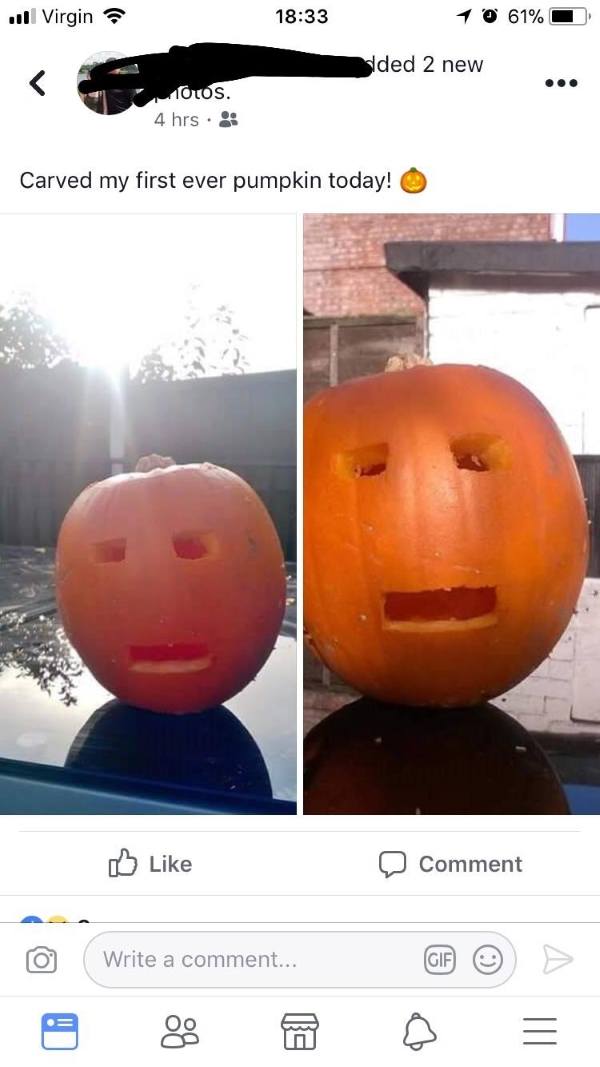**Caption:**

"Today I carved my first-ever pumpkin! 🎃✨ The bright orange pumpkin, now intricately carved, sits proudly on a shiny, reflective black table. In the background, a brick building made of red and white bricks adds an urban charm to the scene. The left photo captures the sunny day with trees casting shadows, while the right photo shows the same setting without the sun. The images are accompanied by interactive icons like a thumbs up, comments section, and share options. Remember, you don't always die from tobacco – sometimes you just lose a lung."